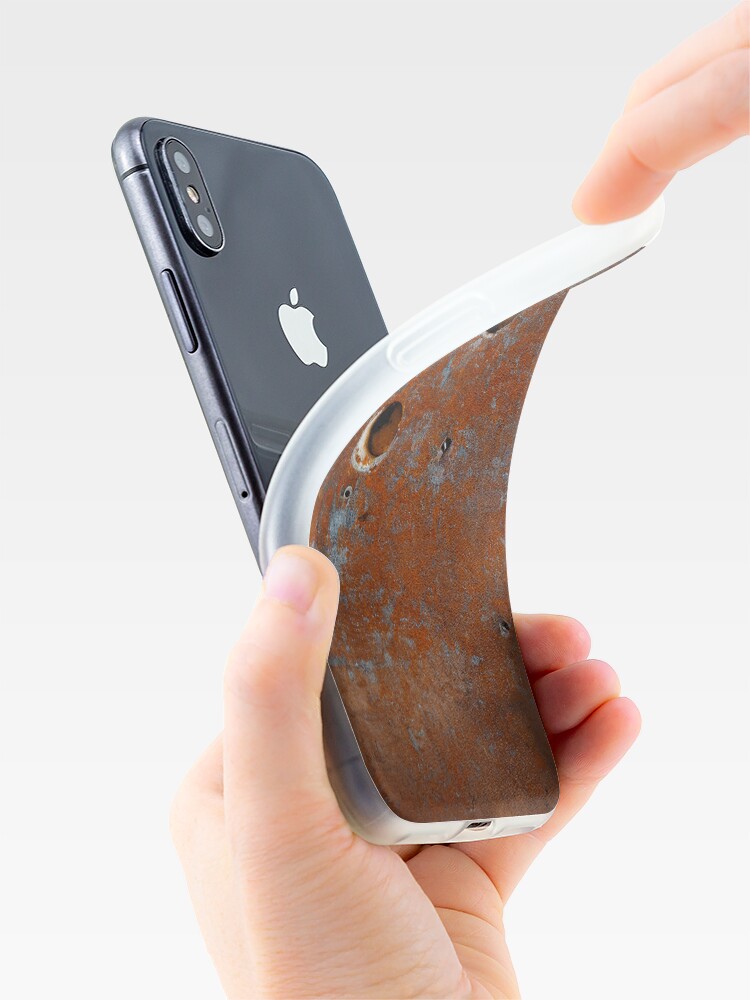An image depicting a Caucasian left hand holding a black Apple iPhone against a very light beige background. The iPhone, shown from the back, prominently displays the white Apple logo. The hand appears to be peeling back an old, protective phone case using a finger from the top right corner of the image, creating a V shape where the phone meets the partially removed case. The back of the case, which has a distressed look, appears mottled with rusty browns and gray, resembling an aged piece of metal with a worn, unattractive texture. This image may be a digital or AI-generated depiction, indicated by the slightly unnatural appearance of the hands and the potentially missing fingers.